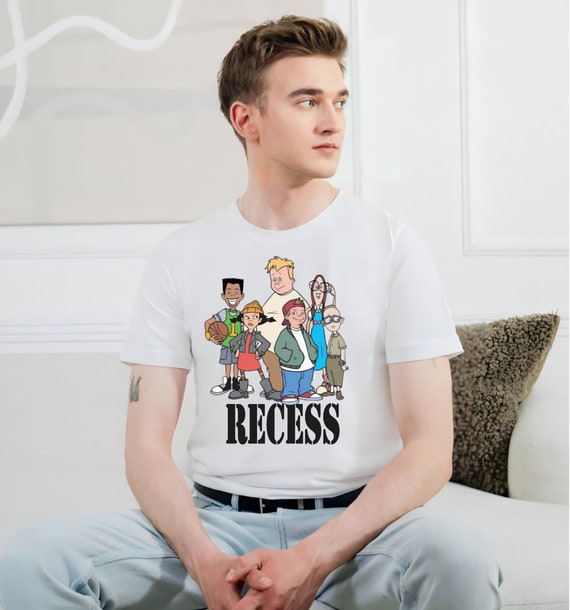A man is seated upright on a white couch, wearing a white t-shirt featuring six characters from the animated show "Recess" above bold black lettering that spells "Recess." The characters include a boy holding a basketball in a green jersey, a girl in a yellow hat, red dress, and gray coat, a larger boy in a white shirt and brown pants, a boy in a red cap, green jacket, white shirt, and blue pants, a tall slender girl in a blue dress with glasses, and the shortest boy in a green outfit with glasses. The man has thick, slightly long brown hair brushed back and sits with his hands clasped, looking off to his left side. He wears light blue jeans with a black belt and has a tattoo on his right bicep, though its full design is not visible. Behind him is a white wall adorned with a subtle gray and white design, and a beige pillow rests on the couch beside him.